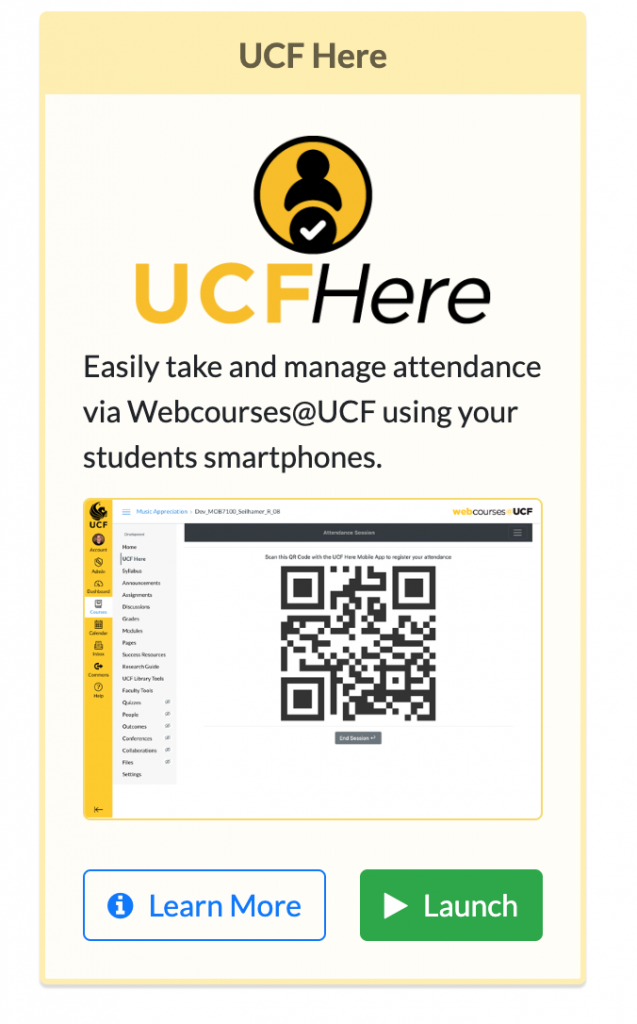This screenshot from an app associated with UCF (University of Central Florida) is displayed against a vibrant yellow background. At the top, the header prominently reads "UCF here." 

Beneath the header, the app logo is centrally positioned on a white background. The logo features an orange circle with a black outline. Inside the circle, there is a graphic of a person above a black circle housing a white check mark. Below this graphical element, "UCF" is written in capitalized orange letters, followed by the word "here" in italicized black text.

The primary text underneath the logo explains the app's functionality: "Easily take and manage attendance via web courses at UCF using your student smartphone." Below this, an inset image demonstrates the user interface. It shows a user selecting an option to retrieve a scannable code, illustrating the process of managing attendance by checking in via smartphone.

At the bottom of the screenshot are two interactive buttons. The button on the left, "Learn More," is outlined with a thin blue line. The text is blue, and an icon of a white eye in a blue circle is positioned to the left of the text. On the right, the "Launch" button is green with white text. It features a white arrow pointing to the right immediately to the left of the word "Launch."